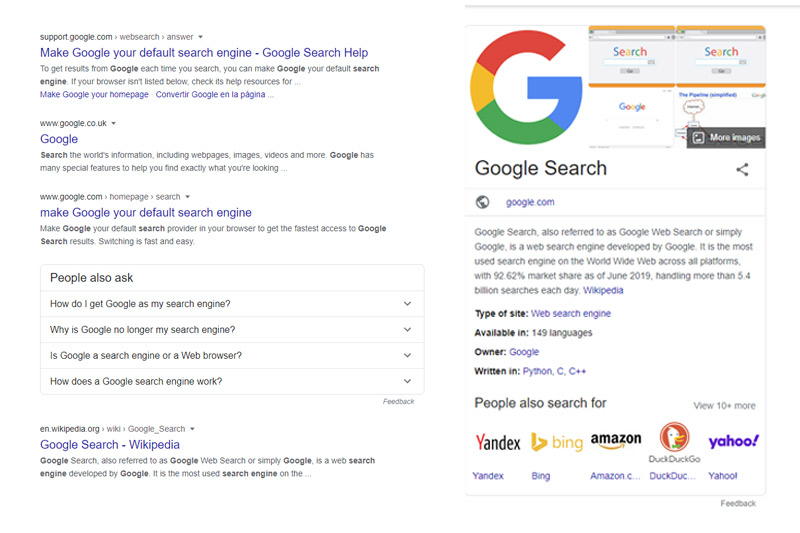The screenshot depicts a search engine results page that strongly resembles Google, despite the logo and parts of the search query being cut off. The search appears to be about how to make Google the default search engine. The first search result reads, "Make Google your default search engine - Google Search Help." Below this, subsequent results include "google.co.uk," "Make Google your default engine," and "Google Search - Wikipedia."

On the right-hand side, there's an informational snippet about Google Search, including a link to "google.com" and a summary from Wikipedia describing Google Search as the most widely used search engine on the web, with a market share of 92.62% as of June 2019, processing over 5.4 billion searches each day. It mentions that the search engine is developed by Google, available in 149 languages, and written in Python, C, and C++. The snippet also lists alternative search engines like Yandex, Bing, Amazon, DuckDuckGo, and Yahoo.

Images shown alongside the search results include historical screenshots of Google’s search pages and the contemporary Google logo, characterized by its iconic multicolored 'G' divided into red, yellow, green, and blue sections.